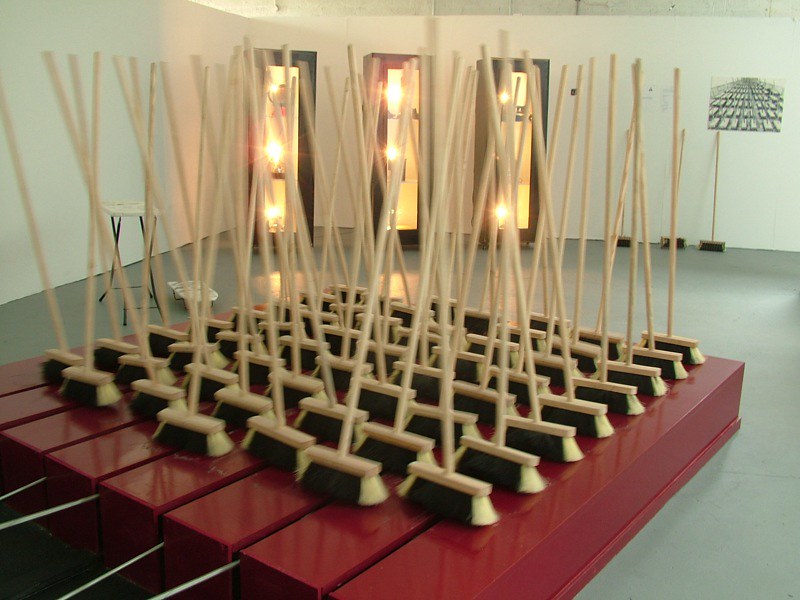In this rectangular photograph, we see a detailed shot of an art exhibit set inside a room with grey concrete flooring and creamy grey walls. The focal point is a series of eight long, six-foot red blocks, each approximately 16 inches high, arranged next to each other. These blocks support numerous upright brooms—each with dark brown bristles that have yellow edges—organized into roughly eight rows of eight brooms each. The brooms are embedded in a track system within the blocks, with metal skewers securing them, and sticks at the ends allowing them to be moved along the track. 

Behind this striking setup, the back wall showcases additional elements, including dustpans, both a tall and a small ironing board, and three lit museum cases whose contents are obstructed by the broom display. There's also an occasional table with a cream top and black legs, and a photograph depicting what appears to be a shelter with people sleeping on cots. The room's overall aesthetic points to a carefully curated art installation, combining everyday objects in a thought-provoking manner.